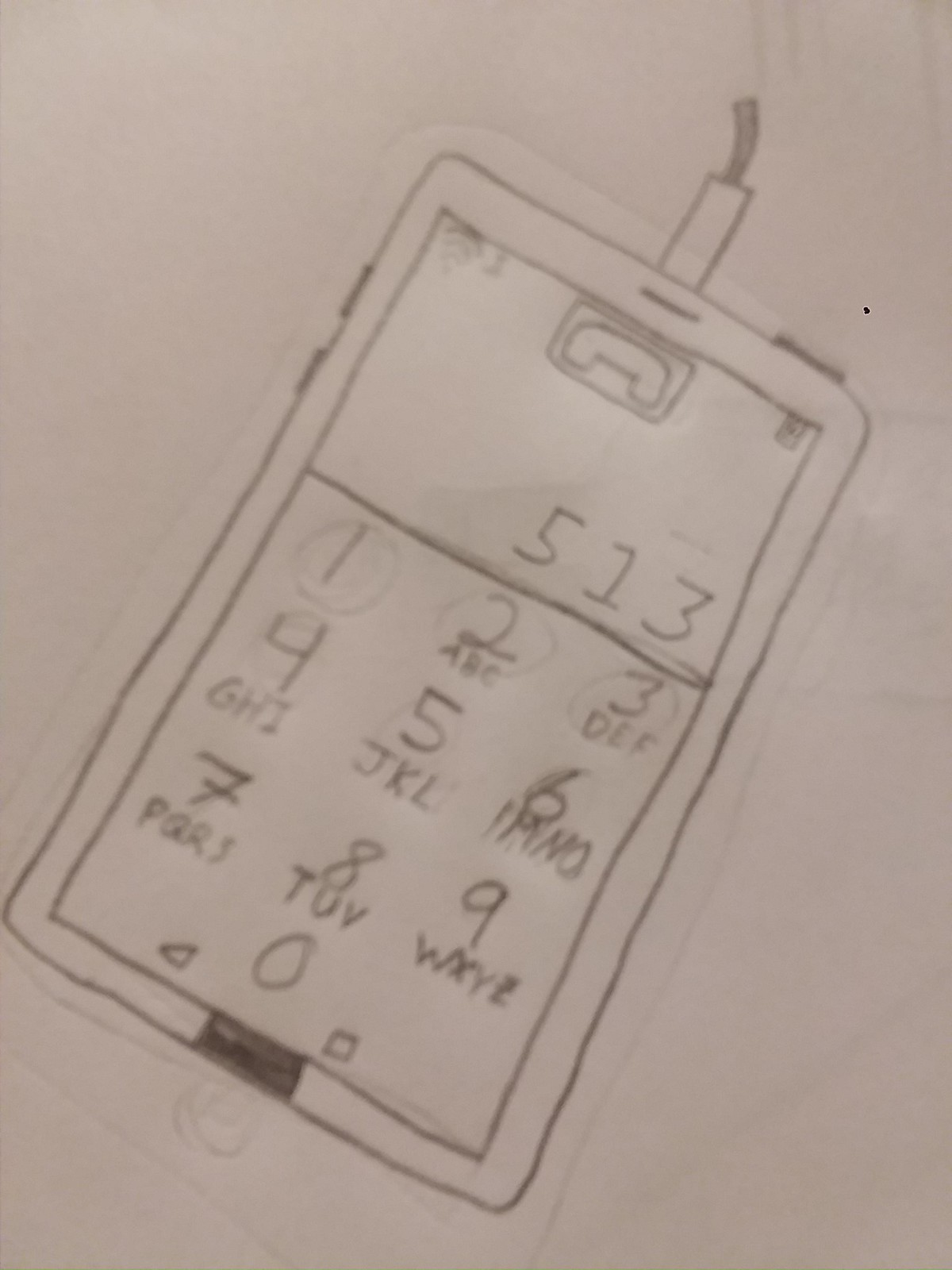This is a detailed pencil illustration of a phone, focusing on the interface and features. The phone's bezel is clearly outlined, framing the internal display. At the top of the interface, there's a small pictogram of a phone positioned horizontally, accompanied by the number "513" beneath it. 

The central section of the interface prominently displays a classic numeric keypad layout, featuring numbers 1 through 9 arranged in three rows of three, followed by the 0 centered at the bottom. Below each number, corresponding letters are visible, as typically found on older phone keypads.

Beneath the 0 key, there are two distinct icons: a left-facing arrow on the left side and a square on the right, possibly indicating navigation or selection keys. Directly below these buttons is a black rectangular section, likely representing a navigation or status bar.

On the top right-hand side of the illustration, a small white spot marks the endpoint of a visible cord, with a black cable extending outward from this point, suggesting a connected handset or headphone. The meticulous details in the illustration capture the essence of a vintage phone design with a blend of functional and aesthetic elements.